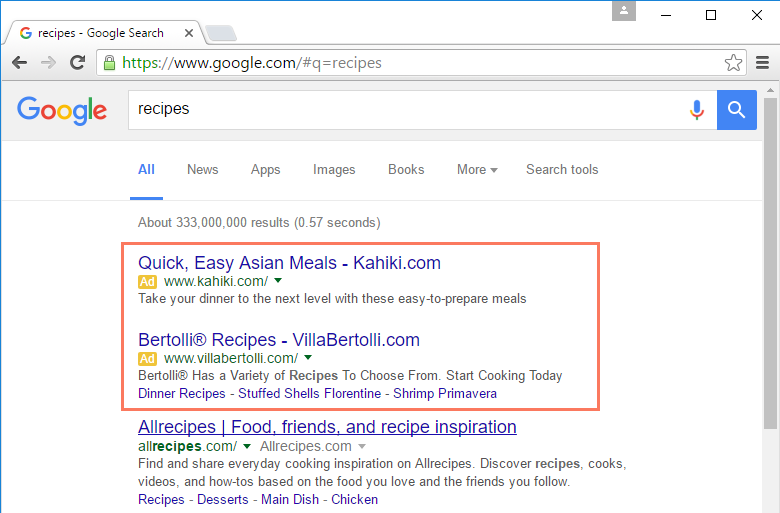A screenshot of a Google search results page for "recipes." At the top, the browser displays standard navigation icons: back arrow, forward arrow, refresh button, and a green padlock indicating a secure connection. The URL bar shows "https://www.google.com/#q=recipes." The Google logo is prominently displayed above the search bar, which contains the query "recipes," accompanied by a microphone icon and a search icon.

Below the search bar are categorized search options: All, News, Apps, Images, Books, More, and Search Tools. The search results indicate about 333,000,000 hits in approximately 0.57 seconds. 

The first result is highlighted with a red box and features "Quick, Easy Asian Meals" from Kahiki.com. The second featured result, from Bertolli.com, is titled "Bertolli Recipes." Additional links include "All Recipes: Food, Friends, and Recipe Inspiration," with categories for Desserts, Main Dish, and Chicken recipes.